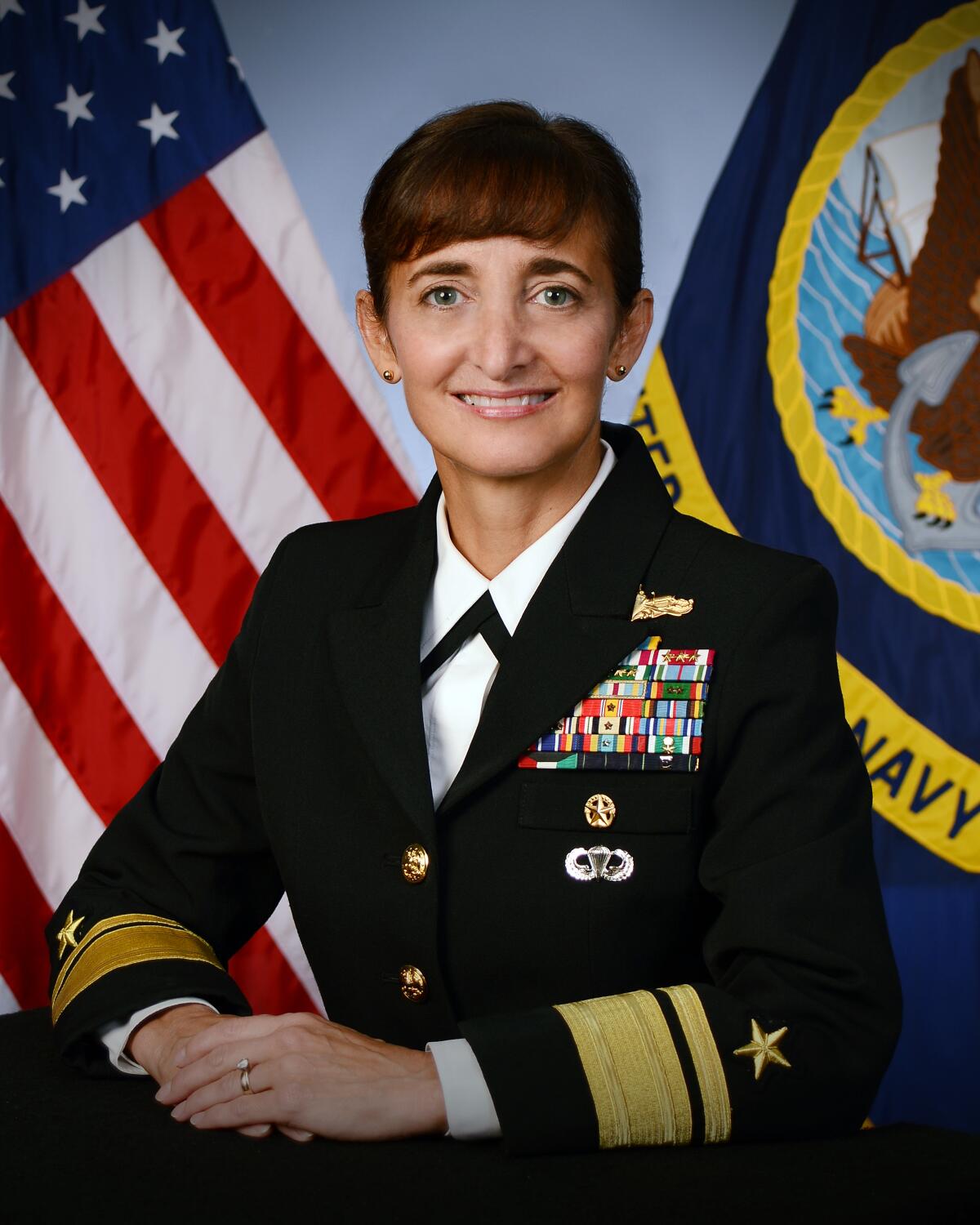The photograph captures a decorated female Navy lieutenant commander in her 40s. She is a white woman with short brown hair cut right above her ears, blue eyes, and modest round gold earrings. Dressed in a full Navy officer’s uniform, she stands at a desk with her hands clasped, displaying a wedding ring. Her uniform features a star on her collar indicating her rank, and her chest is adorned with an impressive array of medals and awards, including a Surface Warfare pin, a parachutist jump school badge, a gold star, a silver medal, and approximately 22 ribbons arranged in 7 rows.

Her sleeves are detailed with gold rings and an embroidered gold star. Behind her, a U.S. Navy flag is visible to the right, featuring an emblem of an eagle standing on an anchor, and an American flag to the left. The backdrop is a blue wall that accentuates the flags, making her decorated presence even more distinguished.